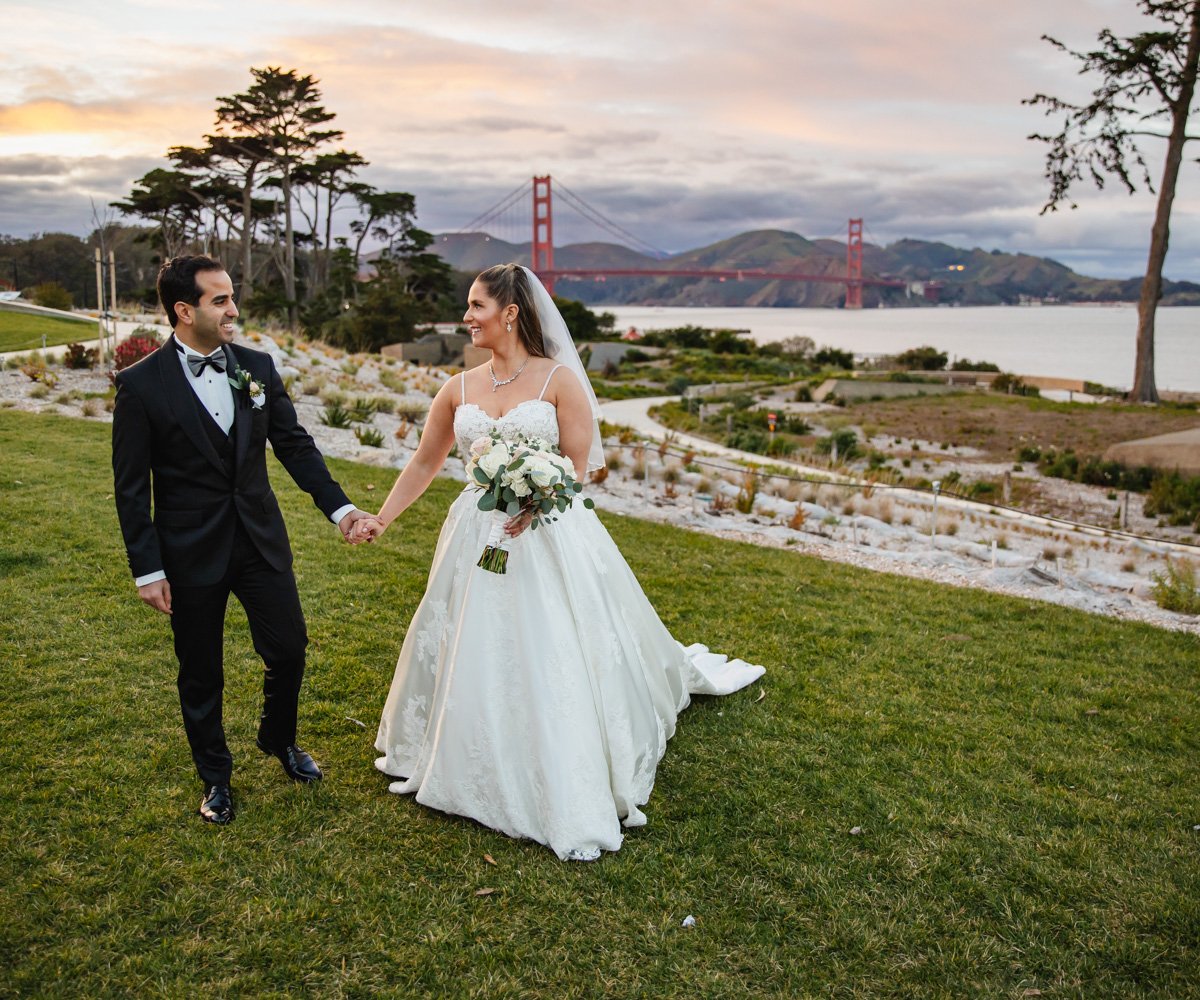This vibrant, outdoor wedding photo captures a joyful moment between a newlywed couple on a gently inclined lawn overlooking the iconic Golden Gate Bridge and the San Francisco Bay. The groom, a Hispanic man adorned in a dark tuxedo with a bow tie and a flower in his lapel, stands hand-in-hand with his bride. The bride, a fair-skinned woman with uncovered, blondish hair, wears a necklace and a spaghetti strap wedding dress that flows elegantly down to her feet. She carries a bouquet of predominantly white roses. Both are smiling warmly as they look into each other's eyes. The background features an expansive view of the bay framed by tall trees and distant mountains, under a sky that's lightly overcast with hints of pink, suggesting a sunset. The photo, clearly professionally taken, is vivid and well-lit, capturing the essence of a perfect wedding day in San Francisco.